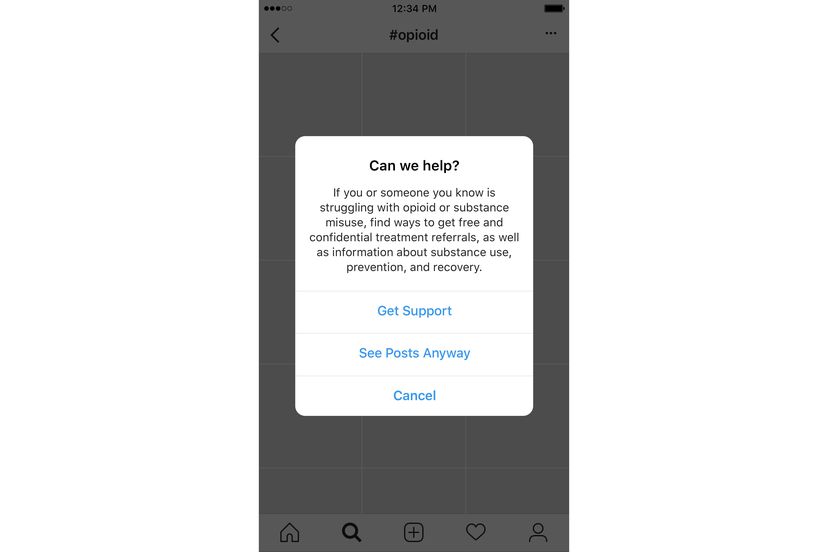The cell phone screenshot, captured at 12:34 PM, presents several interface elements in precise detail. At the top left corner, three black dots sit adjacent to two smaller white dots, indicating some probable notification or settings function. To the right sits a fully charged battery icon in black. Centrally positioned at the top is a left-pointing arrow beside the hashtag #opioid, possibly indicating a navigation option.

Prominently, a popup message appears, reading, "Can we help?" followed by an informative paragraph: "If you or someone you know is struggling with opioid or substance misuse, find ways to get free and confidential treatment referrals as well as information about substance abuse, prevention, and recovery." The popup includes a clickable link labeled "Get Support," with an option to "See Post Anyway." A blue 'Cancel' button provides a means to dismiss the message.

Directly beneath the popup, the screenshot captures a navigation bar featuring a home icon, a search icon, and a heart icon, typical of common mobile application interfaces.